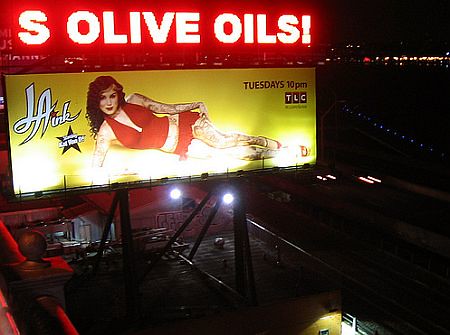The evening scene captures a tranquil cityscape with minimal traffic on the roadways, illuminated by streetlights some of which emit a blue hue. The roadways feature the ghostly trails of passing cars, their lights streaked into long, continuous lines. Dominating the forefront is a towering billboard, supported by sturdy black poles. The billboard's lower half sports a vibrant yellow background with the text "L.A. Link" rendered in white on the left and "Tuesdays at 10 on TLC" in bold black letters on the right. The advertisement showcases a young woman, seemingly named Kat, reclining in a bathing suit and striking a pose in red shoes, displaying her numerous tattoos that cover her from head to toe. Above this scene, the billboard's top section is a striking red, featuring the text "S. Olive Oils" in bold white letters.